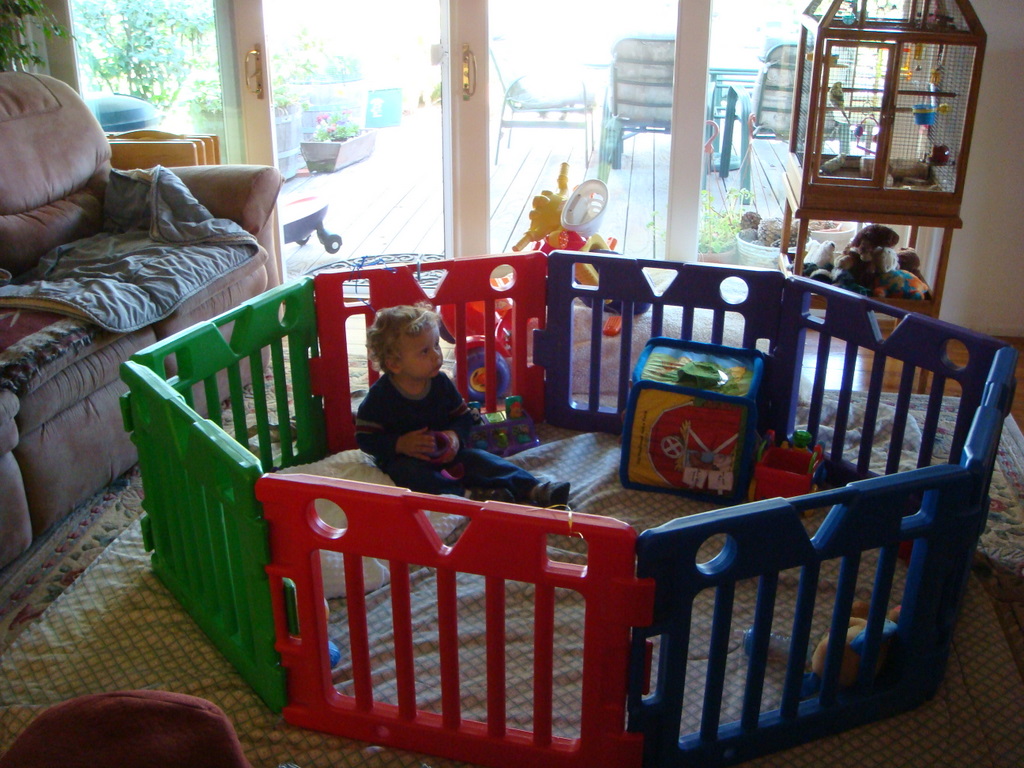In a cozy, well-furnished living room, a colorful playpen made of thick plastic sections stands out in the center. The playpen is circular, assembled from interlocking sections that are blue, red, green, and purple, each featuring vertical bars and various shapes—circles, triangles, and squares—at the top. Inside, a small child, likely around one and a half to two years old with blonde hair, sits quietly on a green and white or gray and white checked mat that lies over a decorative carpet adorned with greens and plums. The child, dressed in a navy blue sweatsuit and small shoes, is gazing towards the right side of the photograph with hands gently cupped together. 

Within the playpen, there's a large, soft block toy, a pillow, a red bucket, and a plush stuffed animal. Adjacent to the playpen, a tan sofa with what appears to be a waterproof pad or possibly a changing pad rests against the left-hand side. The room is somewhat compact, featuring a birdcage in the top right corner containing a bird perched on a horizontal beam, with plush toys on a shelf underneath and a blue watering pail hanging off the side.

Behind the playpen, glass doors with white moldings and metallic handles open up to a deck. The outdoor space includes wooden planks arranged vertically, lounge chairs, and a flower pot with blooming flowers, completing the serene atmosphere of the scene.